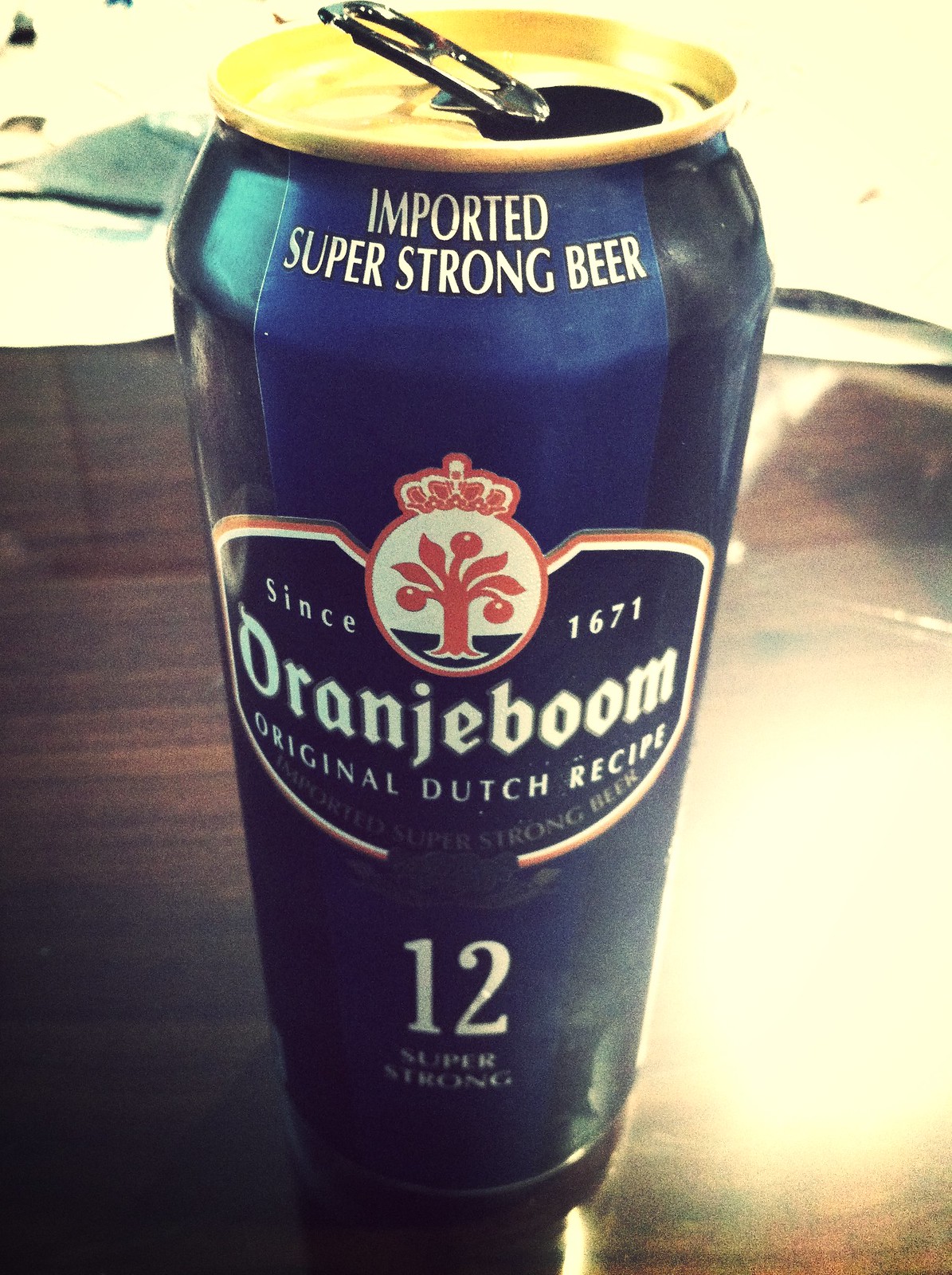The image shows a large, imported can of Orangeboom beer, sitting on a wooden table. The can, which appears to have been opened with some liquid already missing, is distinguished by its striking design: it features a navy blue color on the sides that transitions to a lighter blue in the middle. The top of the can is gold with a black tab. The front of the can prominently displays an orange tree with a crown, alongside an inscription that reads "Since 1671, ORANJEBOOM, Original Dutch recipe, 12 Super Strong." Additional text near the top mentions "Imported super strong beer." The background is predominantly white, which makes the vivid colors of the can stand out even more. The angle of the picture also gives the illusion that the top of the can is larger than the bottom.